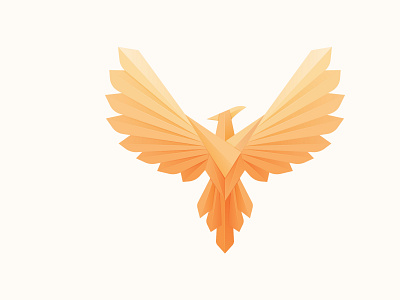This clip art image is a highly stylized illustration of a phoenix, characterized by its wings outstretched in a symmetrical manner. The phoenix, which showcases a gradient color scheme transitioning from pale yellow at the top to a richer orange at the bottom of its tail feathers, is set against an ivory to very pale pink background. The bird has a V-shaped chest and a pointed beak that faces upward and to the right. The tails and wings share similar textures and dimensions, with the wings featuring eight feathers on each side and the tail boasting five feathers. The head is square-shaped, lending an origami-like appearance to the illustration. The design is free of any additional text, attribution, human figures, buildings, vehicles, or other creatures, focusing solely on the mythological bird.